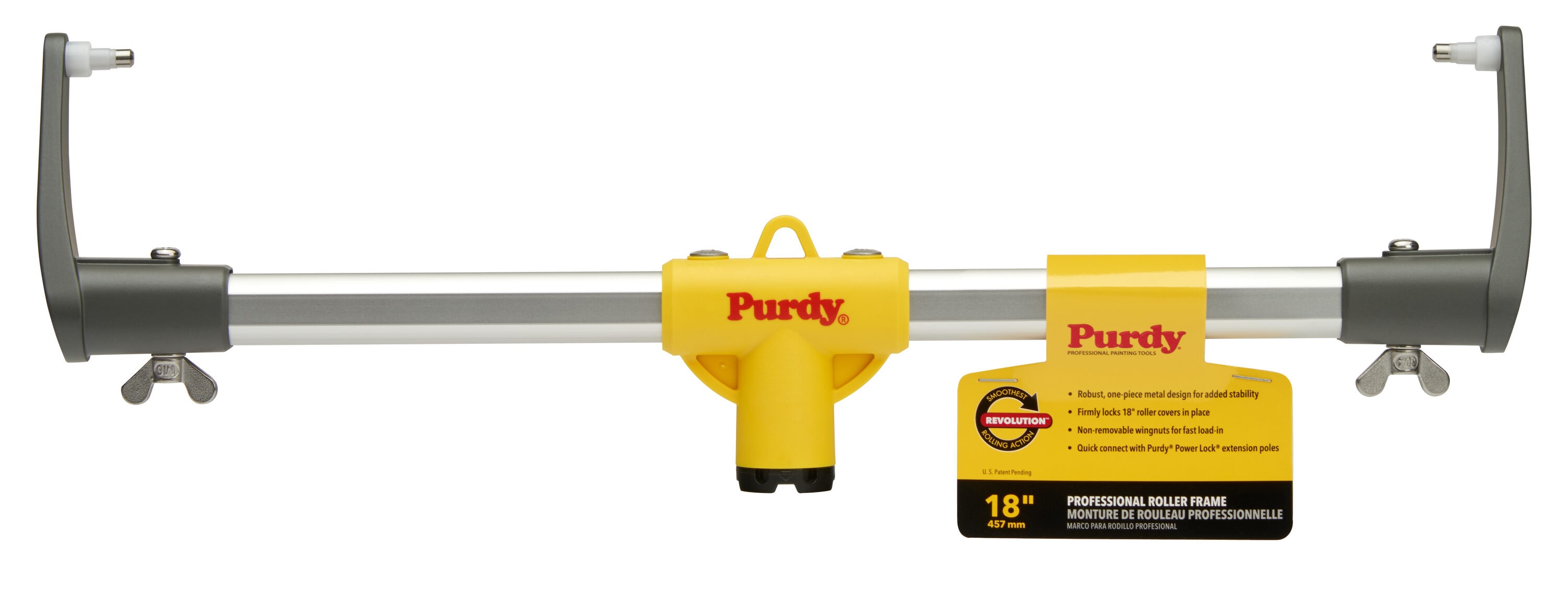The image depicts a professional roller frame by the brand Purdy, prominently displayed against a plain white background. The roller frame, measuring 18 inches (457 millimeters), features a robust one-piece metal design for enhanced stability. It's equipped with non-removable wing nuts that securely lock 18-inch roller covers in place, facilitating fast and efficient loading. In addition to its metallic structure, the frame incorporates plastic components, including two black plastic tips at either end, where it connects and locks, and a yellow plastic piece centrally positioned. This central piece bears the brand name "Purdy" in red text. Attached to the frame is a yellow label detailing its features including compatibility with Purdy Power Lock extension poles. The tag also highlights the product description in various colors: yellow, black, red, and white, ensuring clear visibility of the information provided.